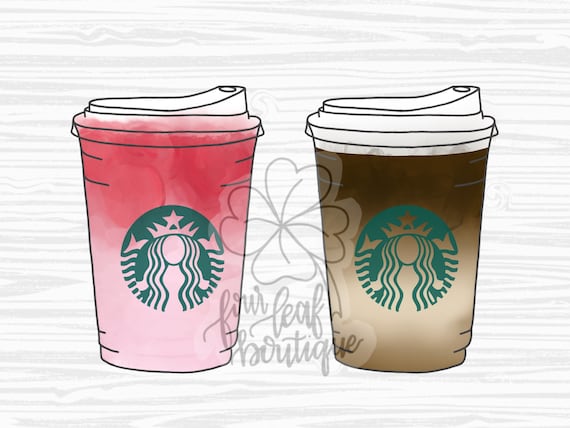The image is a detailed drawing depicting an advertisement for "Four Leaf Boutique." Central to the composition are two identical-sized Starbucks coffee cups, distinguished by their colors and positioned against a softly textured background mimicking the light gray wood grain. The cup on the left transitions from a light pink base to a darker pink top and features a white lid with a sip spout. The Starbucks logo, a green siren, adorns the front. Similarly, the cup on the right exhibits a gradient from light brown to dark brown, also topped with a white lid and the same green logo. Overlaying the center of the image is a light gray outline of a four-leaf clover, beneath which the brand name "Four Leaf Boutique" is inscribed in cursive script. The contrast between the cups—one potentially filled with a pink strawberry beverage and the other with a traditional coffee beverage—along with the minimalist yet sophisticated background, effectively highlights the boutique’s branding.